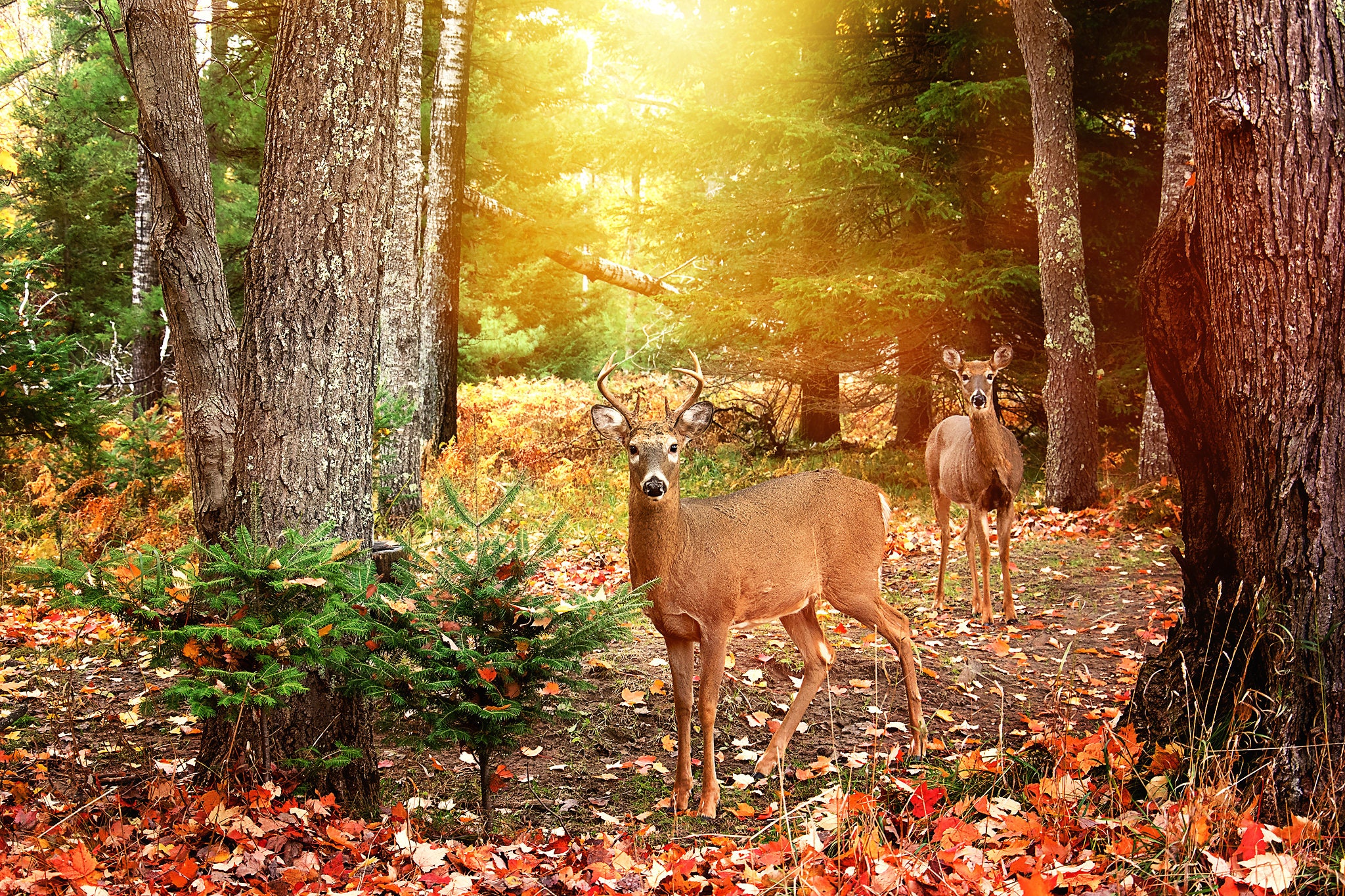This detailed outdoor photograph captures a serene woodland scene featuring two deer standing in a slight clearing amidst a grove of trees. The main focus is a young white-tailed buck, front and center, with small antlers sporting three points each. To the right and slightly behind him stands a doe. Both deer, gazing directly at the camera, have dark eyes, gray and white faces, large brown noses, and medium brown short-haired coats. Surrounding them are large tree trunks with grayish bark, framing the scene. 

To the left of the buck are two small pine trees, and at the base of these trees, green shrubs can be seen. The ground is covered in a colorful array of fallen leaves in hues of orange, red, and white, interspersed with patches of green grass and dirt. In the background, somewhat blurred, are evergreen trees, and bright sunlight streams through the tree canopy, forming a glowing yellow patch in the top middle of the photo. The overall ambiance suggests a tranquil autumnal setting.